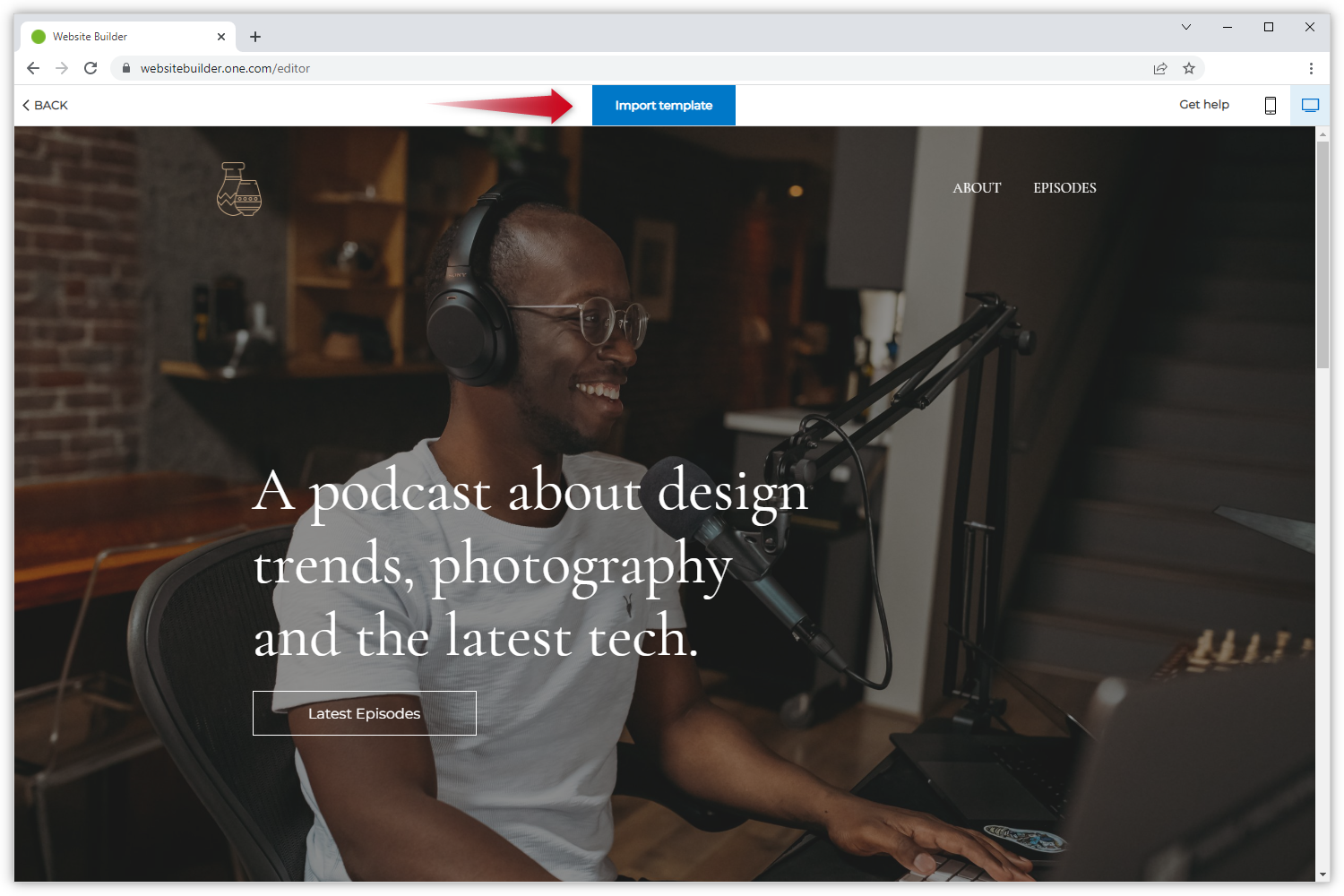The image is a detailed screenshot of a web page. 

At the very top, there is a gray browser interface with an open tab labeled "Website Builder," which has a green indicator on its right side. To the left of this tab, there's a black plus sign for adding new tabs. On the far right, there are the standard browser window controls: a down arrow, minimize button, maximize button, and a close button.

Below this, in the URL bar, are the standard navigation buttons: left and right arrows, a refresh icon, a lock icon, and the URL "WebsiteBuilder.1.com/editor." Next to the URL are additional browser options: a forward button, a star for bookmarking, and a three-dot menu for more options.

On the next line, there's a left arrow labeled "Back." Centrally situated is a large red forward arrow pointing towards the "Import Template" button, which is white text on a dark blue background. On the right side of this line, the words "Get Help" are displayed in black. Additionally, there are icons for making a phone call and a computer monitor. The right edge of the screen contains a gray scroll bar with up and down arrows at its top and bottom.

The main image shows a gentleman wearing headphones and speaking into a microphone, seemingly seated at a keyboard on a desk. To the right of the desk, there is a chess set. A wooden staircase ascends to the right with a nearby wall. In the background, there are shelves and what appears to be a kitchen area, featuring a counter with a coffee pot.

The man has round gold-framed glasses, a bit of a mustache, and is wearing a white short-sleeved t-shirt. He has dark skin and is seated in a black and gray chair. Overlaid on the image, white text reads: "A podcast about design, trends, photography, and the latest tech." At the bottom in a white box, another white text reads: "Latest Episodes."